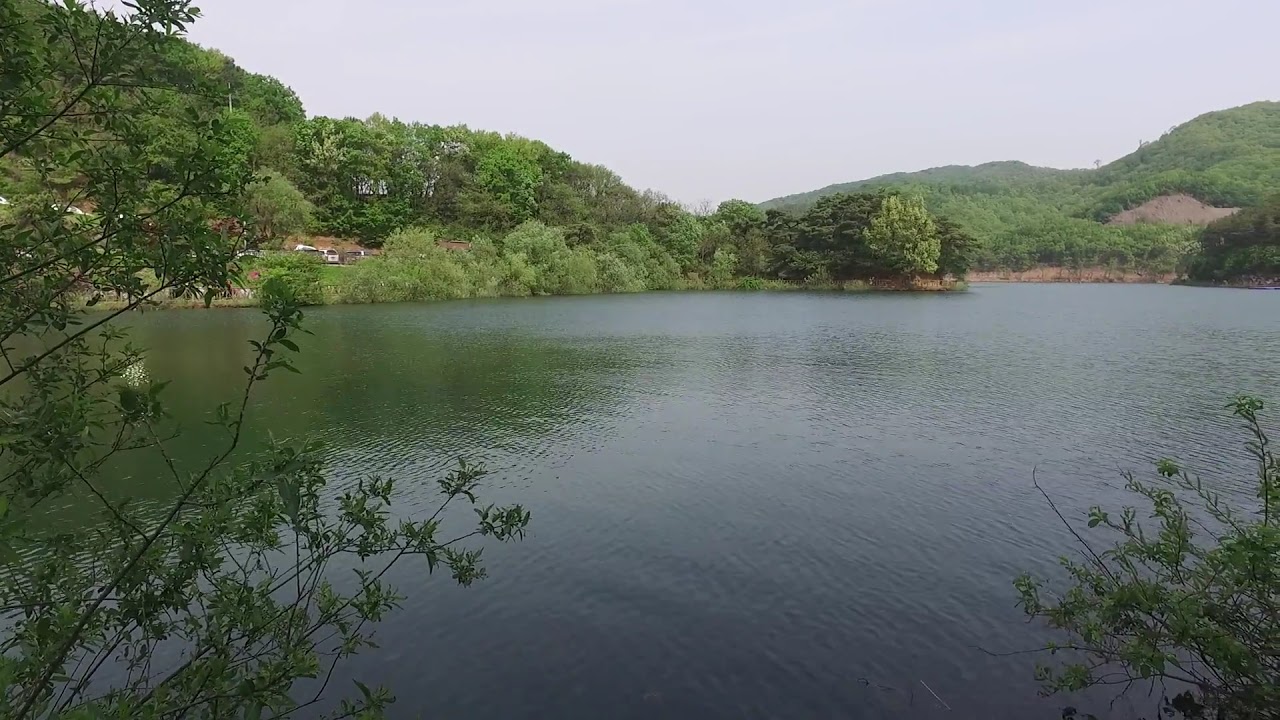This photograph captures a serene lake enveloped by lush greenery. The foreground features silver-blue water, exhibiting gentle ripples that add a subtle texture to the scene. The lake's edge is framed by green bushes and thin branches with green leaves on the left-hand side. Dominating the landscape in the background are rolling, bumpy hills and mountains, all cloaked in various shades of green from trees and bushes. The left side of the image reveals a glimpse of civilization with a few cars parked, but otherwise, the scene is a tranquil natural setting. The sky above is a light gray, cloud-covered expanse, contributing to the overall calm and dull ambiance of the day. The pristine, clear water and vibrant greenery make for a picturesque view that could easily be turned into a captivating jigsaw puzzle.